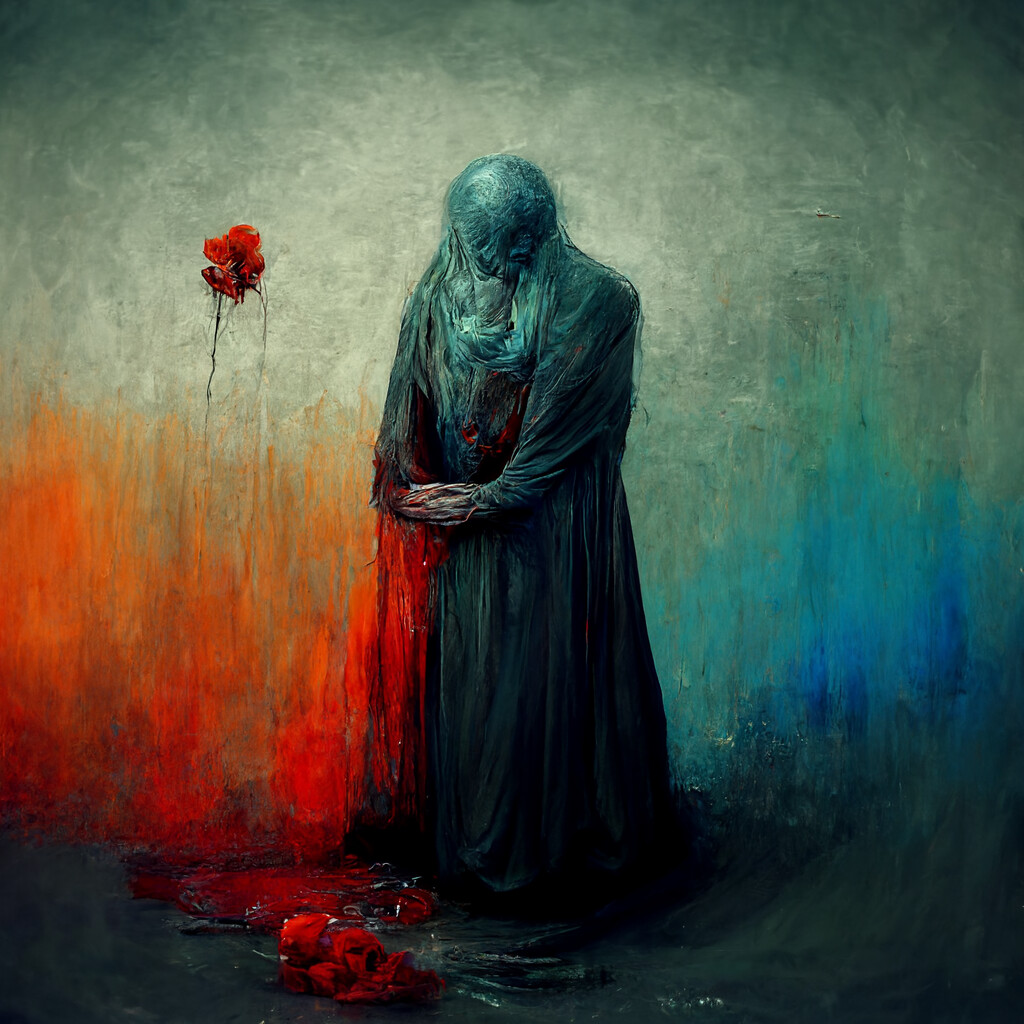The painting depicts a cloaked, faceless figure standing solemnly in the center, dressed in a long, dark robe. The figure's right arm is absent, with a gushing waterfall of blood cascading down to form a crimson puddle on the floor. Surrounding the figure are red roses, some scattered on the ground among shards of a broken vase, adding to the scene's somber mood. One prominent rose is encased in the wall to the left of the figure. The background transitions through various colors; on the right, shades of green and blue swirl together, gradually shifting into a dark gray at the top. The left side of the painting features orange hues that meld into the blood-like substance encroaching the scene, enhancing the dramatic contrast. The overall atmosphere is dark and disturbing, suggesting themes of loss and heartbreak.